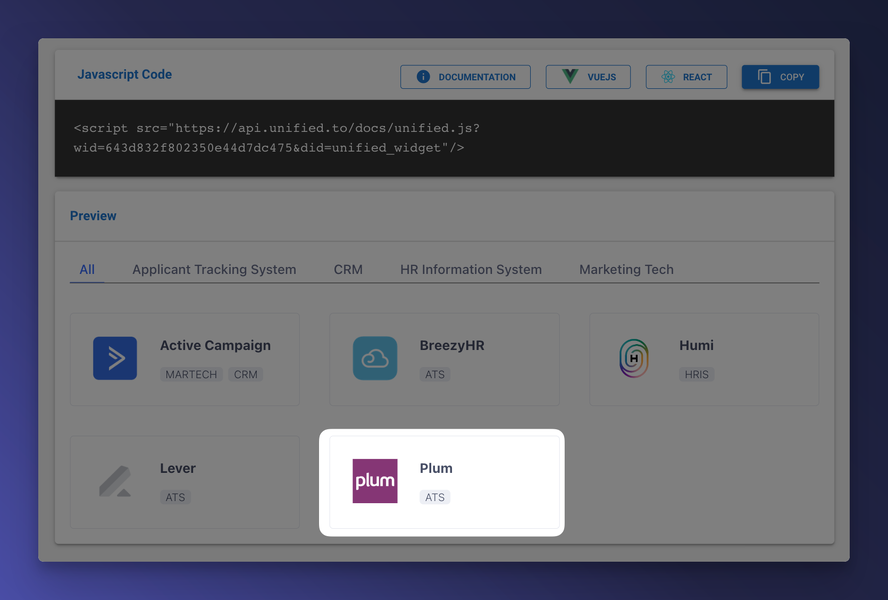Here's a detailed descriptive caption for the image:

---

A screenshot of a software application's interface is depicted. The main focus of the screen is a darkened, grayed-out background, with a highlighted section near the bottom. This highlighted part indicates that the item "Plum ATS" has been selected. To the left of this selection is a small logo, and to the right is the text "Plum ATS."

At the top of the image, the screen displays the words "JavaScript Code," while the right side features documentation related to the code. This documentation seems to cover different frameworks, namely Vue.js and React.js, both associated with JavaScript.

There is a distinct "Copy" button, which allows users to copy the displayed JavaScript code. This code is shown on a black background, effectively distinguishing it from the rest of the interface, which generally has a white but now grayed-out background. 

Below the JavaScript code section, there's a "Preview" area that likely shows a visual representation or output of the written code. 

Finally, the very bottom of the image contains a series of tabs, which include titles such as "Applicant Tracking System," "CRM," "HR Information System," "Marketing Tech," and "Active Campaign." Other visible tool names in the tabs are "Breezy HR," "Humi," "Lever," and "Plum."

---

This detailed caption provides a clear and comprehensive description of the screenshot, making it easier for readers to understand without needing to see the image.